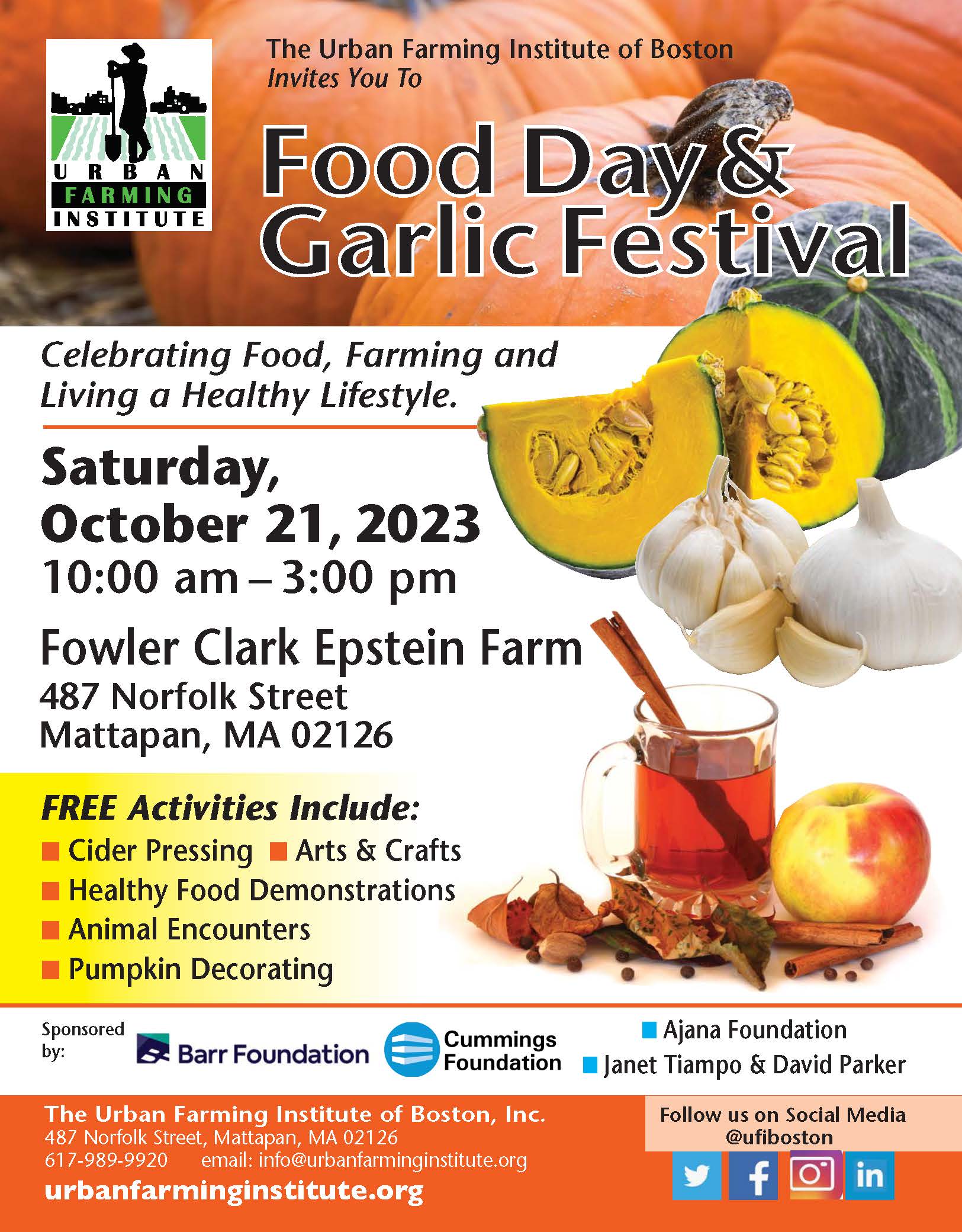The Urban Farming Institute of Boston is hosting a vibrant and informative Food Day and Garlic Festival, emphasizing a celebration of food, farming, and healthy living. The colorful advertisement features a background of pumpkins, squash, garlic, apple cider with a cinnamon stick, and other autumn-themed vegetables and spices. The event, held at the Fowler Clark Epstein Farm, located at 487 Norfolk Street, Mattapan, Massachusetts, will take place on Saturday, October 21st, 2023, from 10 a.m. to 3 p.m. Attendees can enjoy free activities such as cider pressing, arts and crafts, healthy food demonstrations, animal encounters, and pumpkin decorating. The ad highlights that the event is sponsored by the Barr Foundation, Cummings Foundation, and the Adjana Foundation. For more information and social media links, visitors are directed to urbanfarminginstitute.org.